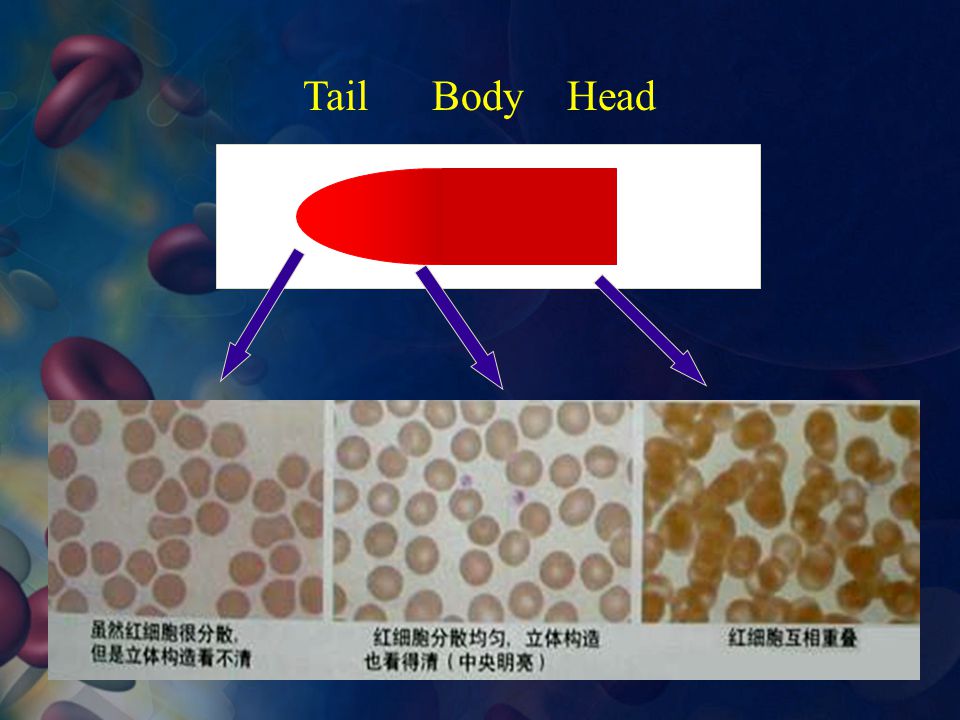The image is a detailed scientific illustration resembling a PowerPoint slide, characterized by a predominantly blue background that transitions from a lighter blue on the left to a darker shade on the right. The left side of the image features oval, three-dimensional, purple disks against the lighter blue portion. Central to the image is a white rectangle that contains a red, bullet-shaped figure oriented to the left. At the top of the image, yellow text reads "Tail, Body, Head," with each word capitalized. 

From the red bullet shape, three blue arrows extend downward. The first arrow points down and to the left, while the other two arrows point down and to the right. These arrows direct attention to three distinct squares, each containing what appear to be high-resolution photographs of microscopic slides showing pinkish, round blobs, likely bacteria or cells, viewed under a microscope. Each of these images showcases different cells or molecular structures, corresponding to the labelled sections "Tail," "Body," and "Head." Below each square, black text in Japanese or Chinese characters provides further description or annotation.